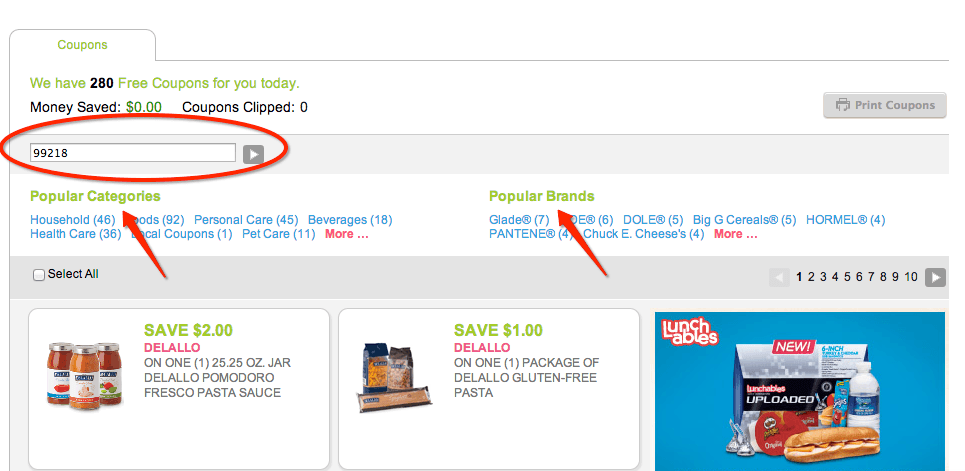The image is a screenshot of a coupon website, specifically focused on offering free coupons. At the top of the page, there's a green-highlighted tab labeled "Coupons." Right beneath this tab, in green text, it states "280 free coupons today," with the number "280" in black. Below this, there's an informational line displaying "Money saved: $0" and "Coupons clipped: 0," giving a quick overview of the user's current activities.

On the far right of the top information bar, there's an option labeled "Print Coupons" accompanied by a small printer icon. Directly below, there's a filled-out field featuring the numbers "99218" with a play button to its right, possibly indicating a captcha or verification step.

The main content section underneath these elements is divided into "Popular Categories" and "Popular Brands," showcasing various items under each section. Towards the bottom of this main area, there's pagination available, allowing the user to navigate through pages 1 to 10 either by clicking on individual numbers or using arrows to cycle through.

On the bottom left, under the section titled "Popular Categories," there is a "select all" checkbox option that currently remains unchecked. In this area, a few specific products are listed:

1. The first product offers "Save $2 on de la low."
2. The second product offers "Save $1 on de la low."
3. The third appears to be an ad for "Lunchables Uploaded," which stands out due to its different, more promotional format compared to the adjacent products.

The overall color scheme of the webpage is predominantly green and white, with hints of blue and red to highlight various elements.